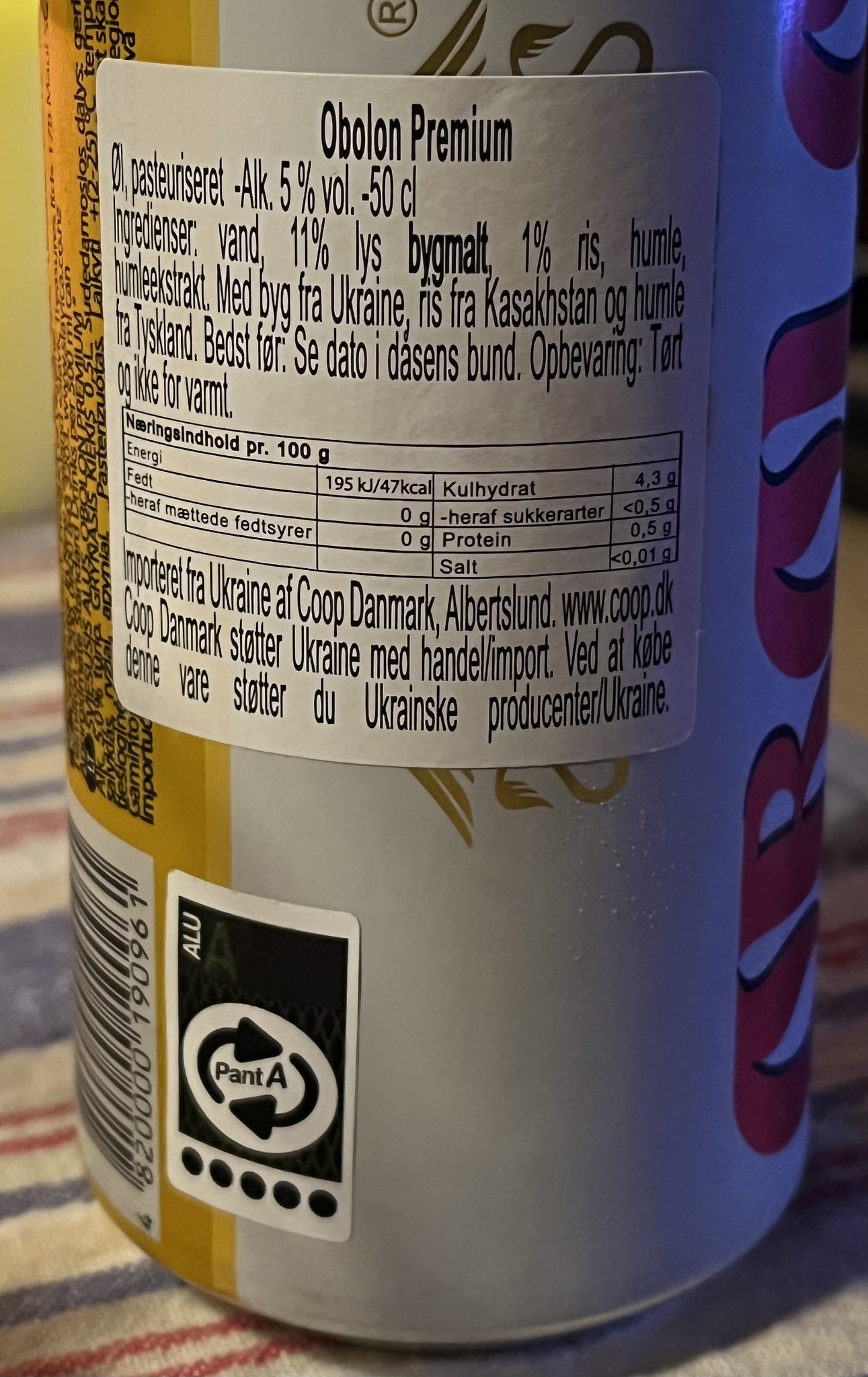The photograph, taken in portrait mode, captures a tall can with a visible label. The can bears the name "Obolon Premium" prominently on its back, alongside smaller text in what appears to be a European language, likely from the Ukraine region. This is suggested by recognizable words such as "Ukraine" and "Co-op Denmark" near the bottom of the label. The can's full information, including ingredients, is written in the same foreign language, though much of the text is obscured by the angle of the can and a partially covering sticker.